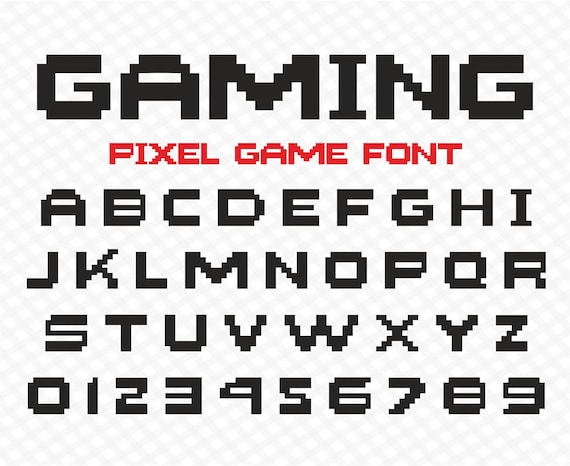The image showcases a digital-style, text-based print designed to mimic the aesthetic of 1980s arcade video games. The square image features a background of white squares intersected by horizontal and vertical lines, forming a subtle grid pattern that fades towards the bottom of the image. The centerpiece is the text, which is entirely in all-caps pixelated, blocky font reminiscent of classic video game graphics. At the top, "GAMING" is prominently displayed in bold black pixels. Directly beneath it, in a smaller but similarly pixelated font, the text "PIXEL GAME FONT" appears in bright red. Following this, the entire alphabet from A to Z is arranged in three horizontal rows: A-I, J-R, and S-Z. Below the alphabet, the numbers 0 through 9 are displayed. This meticulously designed piece, with its pixelated characters composed of tiny rectangles or squares, evokes the charm and nostalgia of early video game typography.